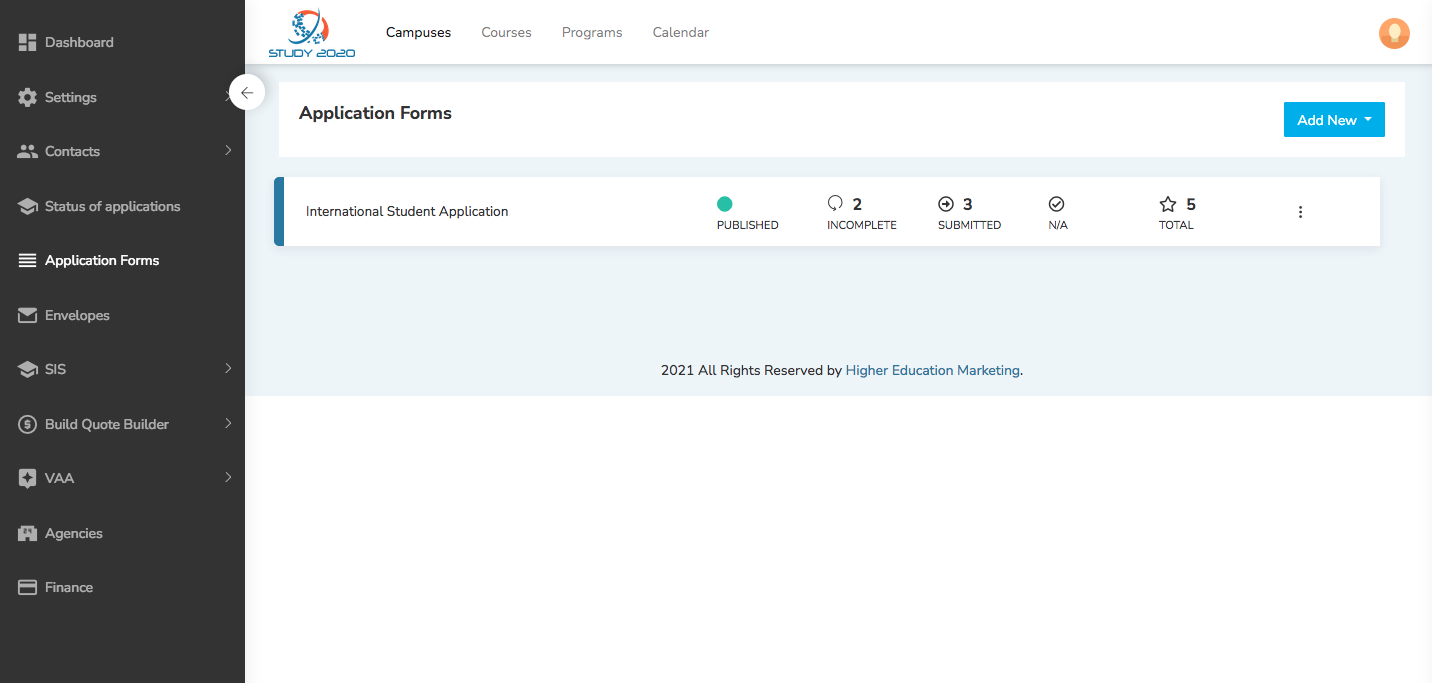This screenshot is taken from an application dashboard belonging to a website identified by its unique logo, labeled "Study 2020" beneath it. The view showcases the user interacting with the "Campus" section of the interface, specifically highlighted as they work on submitting an international student application. The application is visibly incomplete, with two text fields left unfilled. Out of five required submission fields, only three have been completed, while two remain pending completion. Adjacent to this, a green circle icon with the word "Published" indicates a status or notification within the application.